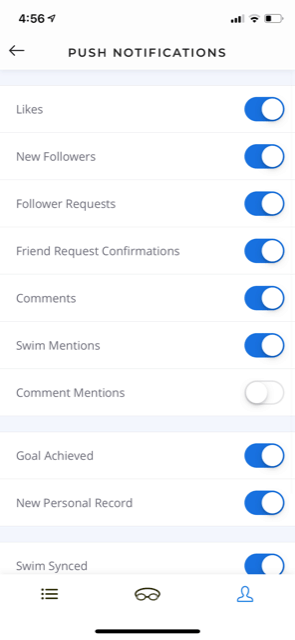This is a detailed mobile screenshot depicting the push notification settings of an app. The screenshot was captured at 4:56, as indicated in the top-left corner. There is a paper airplane icon next to the time, though its specific function—possibly notifications or location—is unclear.

On the top-right corner, there are standard status icons showing cellular service signal, Wi-Fi signal, and battery life, which appears to be approximately 25-30% charged.

The main header at the top of this settings screen reads "Push Notifications" in bold black text on a white background, with a black arrow on the left side for navigating back. Below this header, the screen is composed of multiple sections, each divided by gray lines against a light gray background. The sections contain rows with white backgrounds.

Each row lists different notification options along with their corresponding toggle switches on the right side. In the first section, the options include:
- Likes
- New followers
- Follower requests
- Friend requests
- Confirmations
- Comments
- Swim mentions
- Comment mentions (the only option toggled off)

The second section features:
- Goals achieved
- New personal record

The third and final section has a single option:
- Swim synced

At the bottom of the screen, there are various icon buttons for additional settings within the app. All toggle switches are enabled except for the "Comment mentions" toggle, which is in the off position.